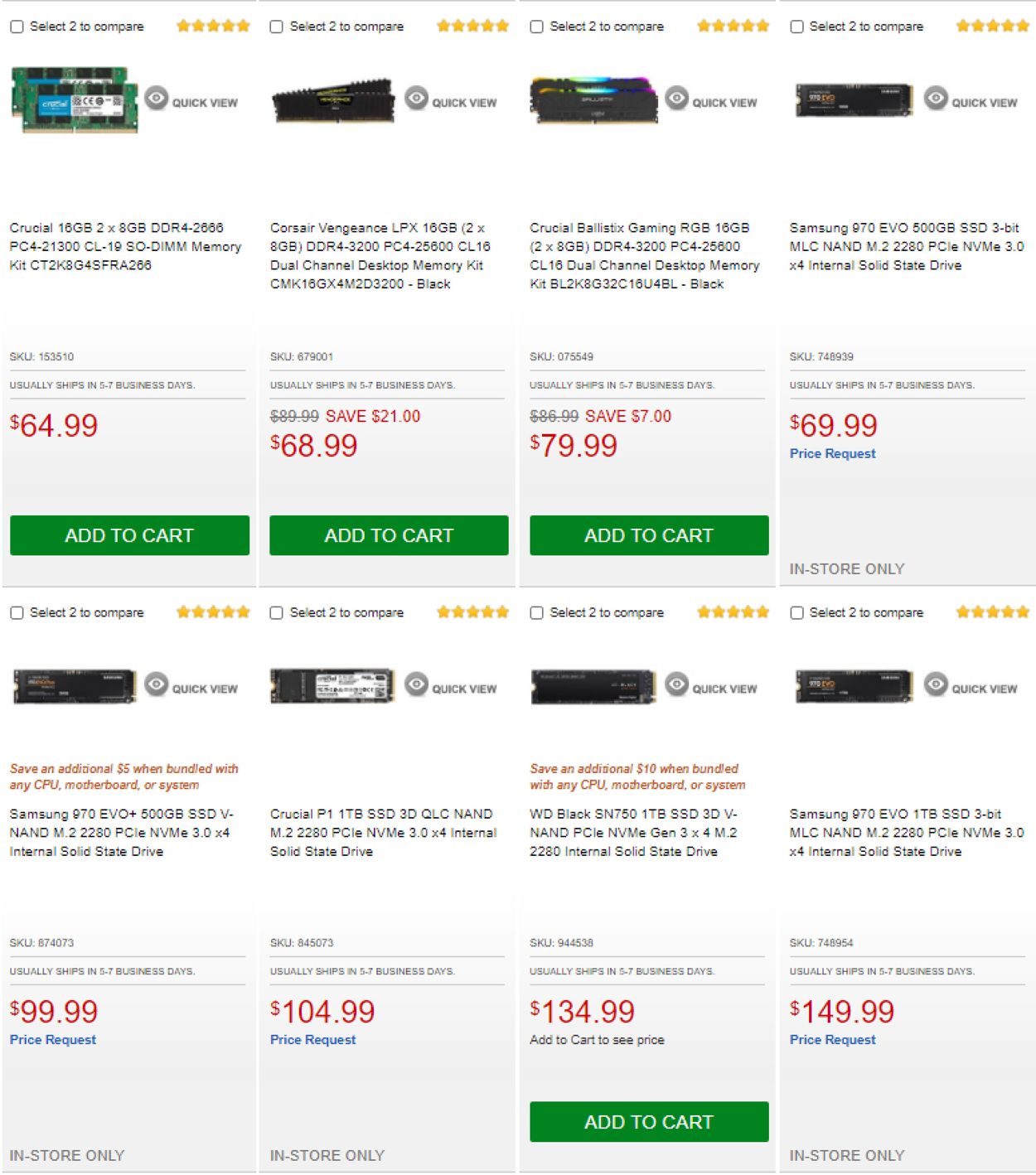The image is a screenshot from a computer parts e-commerce website featuring eight different product listings for RAM modules. The listings are arranged in two rows, with four products in the top row and four in the bottom row. Each product listing features a 'Select to Compare' checkbox in the top left corner and a star rating in gold in the top right corner. Directly below the star rating is an image of the respective RAM module.

Beneath each image is a text description detailing the specific type of RAM, its capacity in gigabytes, the number of modules included in the kit, and the RAM type. Following the descriptive text is the SKU number, which is used for tracking inventory, and the estimated shipping time for the product. The price for each RAM module is prominently displayed in red below the shipping information.

Below the price, each listing has either a green 'Add to Cart' button or gray text indicating 'In-Store Only' availability. In the first row of listings, the first three products have an 'Add to Cart' button, while the last one is marked 'In-Store Only.' In the second row, the first two listings are marked 'In-Store Only,' the third listing has an 'Add to Cart' button, and the fourth listing also indicates 'In-Store Only' availability.